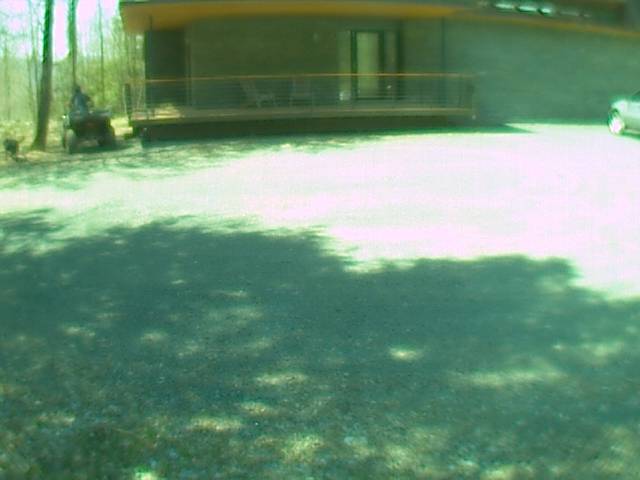This high-contrast photograph captures the front view of a grayish house nestled in a wooded area. The dominant green hues create a vivid backdrop, while the lighter colors are washed out, presenting a stark white in places. Central to the image is a wooden patio extending from the house, adorned with two wooden chairs. The house features a notable back door that opens onto this inviting outdoor space. To the left of the house, an ATV is visible with a person seated inside, implying a ready-for-adventure vibe. To the right, a garage stands with a silver car parked in front, hinting at the daily life of the inhabitants. In the background, tall trees frame the scene, reinforcing the tranquil, nature-immersed setting.